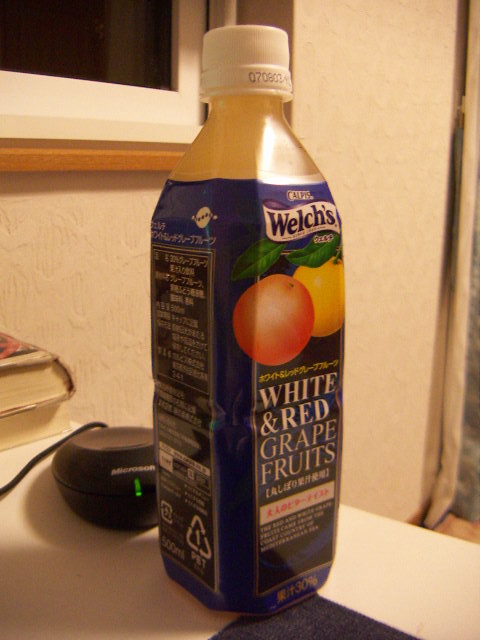The image depicts a rectangular plastic juice bottle with a white cap, prominently placed on a white table that appears to have a black cloth underneath the bottle. The bottle, which is yellowish due to the juice inside, features a predominantly blue plastic-coated label. The label shows images of an orange and a yellow citrus fruit, likely depicting grapefruits, accompanied by green leaves. It has both English text that reads "White and Red Grapefruit" and some Chinese or Japanese inscriptions. The bottle displays the brand name "Welch's" in white on a blue background. Additionally, on one side of the label, nutritional information and ingredients are listed in black squares. Behind the bottle is a wired microphone device with white writing and a green light at its center, connected by a black cord that trails off to the bottom left of the image. Two books are stacked behind the device, and above them is a window with a wooden windowsill. The scene denotes a casual yet cluttered desktop setup, further reinforced by the presence of what appears to be a Microsoft mouse.